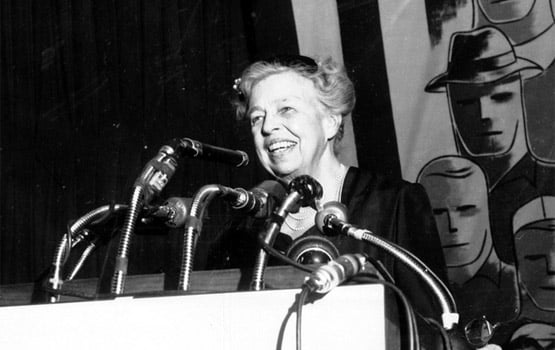In this black and white photograph, Eleanor Roosevelt is depicted smiling warmly as she stands at a wooden lectern with a white surface attached to its front. She is elegantly dressed in a loose black dress, complemented by a small black hat atop her hair, which is pulled up. A delicate pearl necklace adorns her neck, adding a touch of sophistication. In front of her are six upright microphones, capturing her speech. The backdrop is a stark black, accentuating her figure, and to the right hangs a white banner with a black border. This banner features a simplistic, stylized drawing of a crowd with impassive faces, adding a unique, vintage touch to the scene.